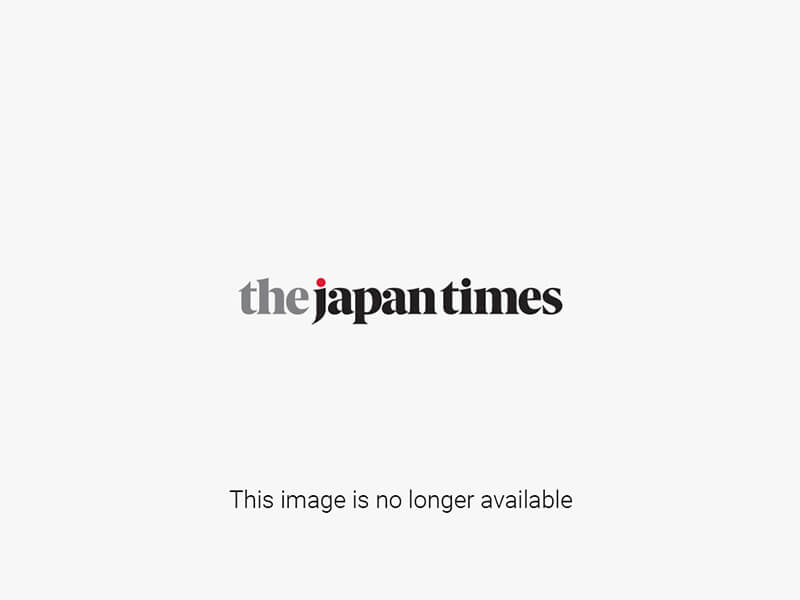This detailed image captures two Asian women, likely tourists, standing in what appears to be an airport, indicated by the high overhead lights and an arrival and departure board behind them. Both women are showcasing their passport books filled with visa stamps, proudly displaying their travel history. The woman on the left is wearing a brown hat, a yellow shirt, and is holding her passport in her left hand. She has short hair tucked under her hat and is looking directly at the camera with a neutral expression. Her passport features numerous stamps, including two with black rectangles. The woman on the right, who is smiling, has short, curled brown hair ending above her ears and is wearing a dark shirt. She holds her passport with both hands. While the details on the passports aren't legible, it's evident that they've traveled extensively. An additional detail captured is a possible mask to the right of the screen, enhancing the contemporary context of the scene.